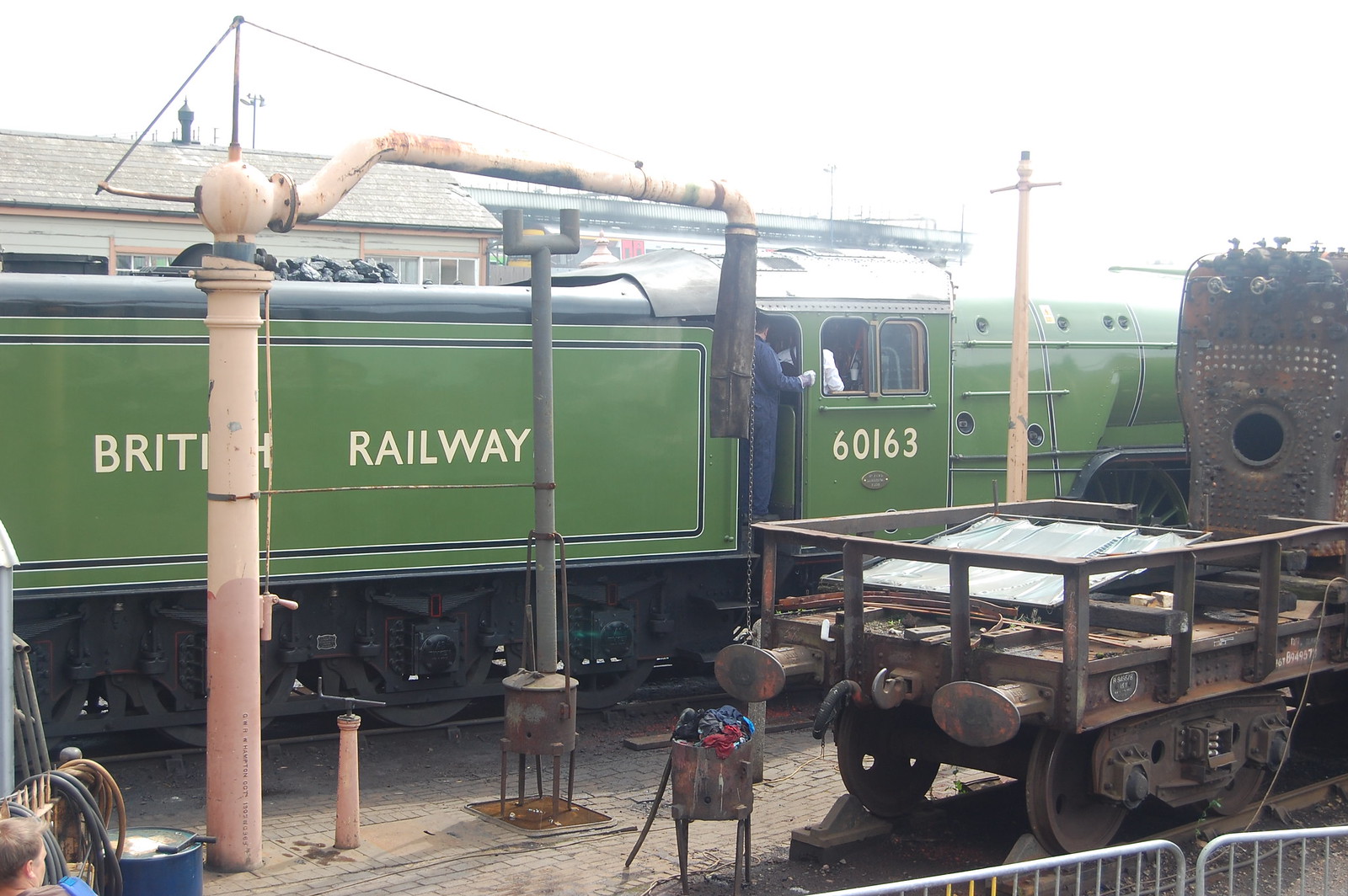In this detailed and nostalgic image, the centerpiece is a stunning British Railway train, captured in what looks to be a 1950s-era setting. The striking green train bears the inscription "British Railways" in white lettering, though the word "British" is partially obscured by a beige pipe. The engine number, 60163, is clearly displayed on the door where an engineer stands, adding a human element to the scene. The train is at rest in a station or depot, and the daylight illuminates the scene with natural brightness. To the right of the main train car, there's a rust-colored brown service truck designed for rail use, identifiable by its turret front and flatbed back, used to push or pull powerless cars. On the lower left side, a young boy peers curiously around equipment that includes a hose-wrapped apparatus and a blue metal barrel. A tall, bending beige lamp post stands in front of the train, and other green railway cars are visible in the background, accompanied by what could be a waiting area or a train station.